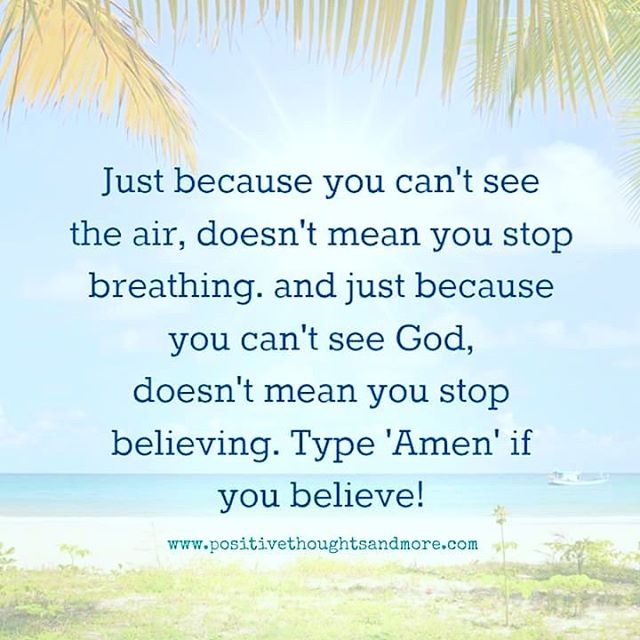This square image features a serene tropical scene with a light blue sky and white cloud outline in the top right corner. Palm leaves hang down from the top edge, framing the image. In the center, a bright sun with radiant rays illuminates the scene, casting a warm glow over the ocean in the background. The foreground showcases a picturesque shoreline adorned with white sand, grassy areas, and a tall flower stem. A small boat is visible in the crystal clear blue water. Overlaid on this washed-out scenic backdrop is a motivational text in dark blue, which reads: "Just because you can't see the air doesn't mean you stop breathing. And just because you can't see God doesn't mean you stop believing. Type 'Amen' if you believe!" Below this text, in a different shade of blue, is the URL: www.positivethoughtsandmore.com.